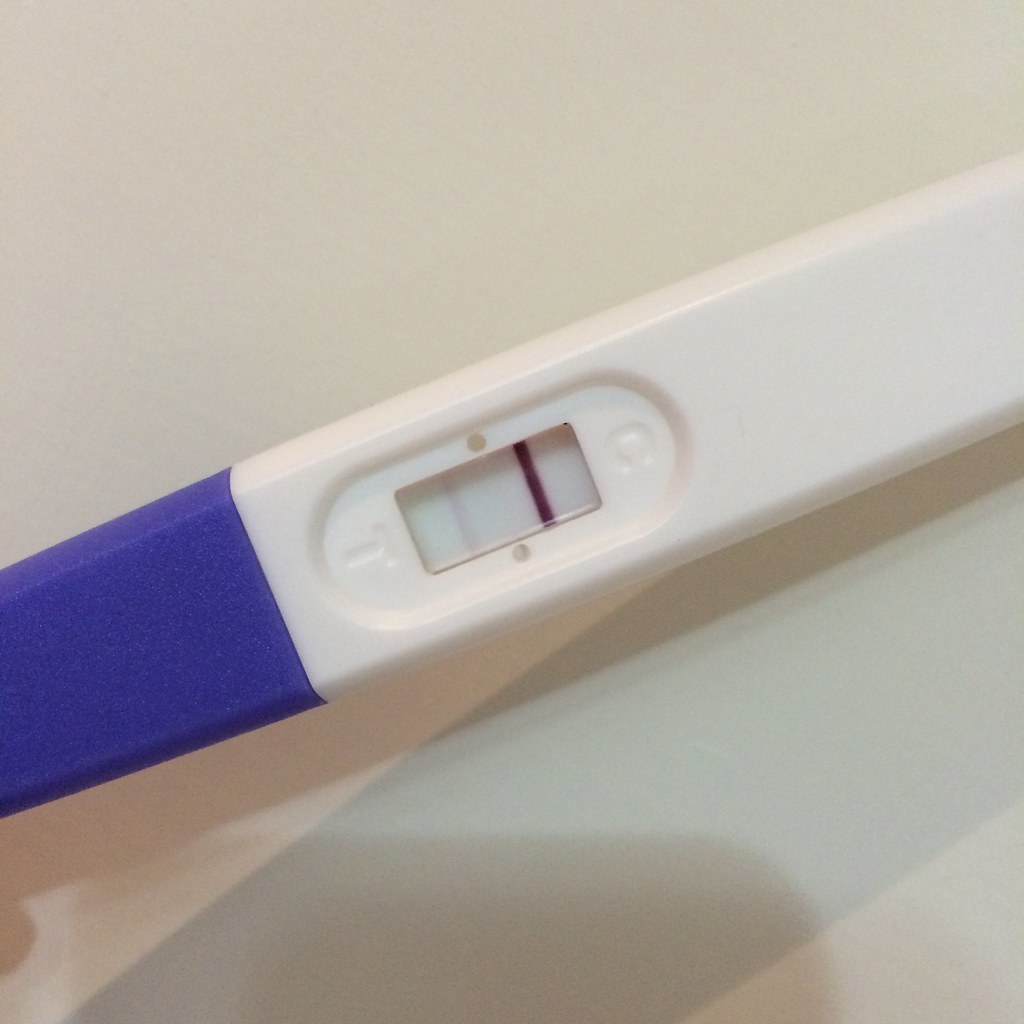This image is a close-up photograph of a pregnancy test placed against a white background. The test, predominantly white, features a rectangular body with a distinct blue handle visible on the left side. The central focus of the test is an oval-shaped inset located just to the right of the blue handle. Within this oval, there is a small rectangular screen displaying two lines: a darker red line on the far right and a very faint line on the left. The right side of the rectangle within the oval is marked with an imprinted letter "C," while the left side, adjacent to the faint line, is marked with the letter "T."